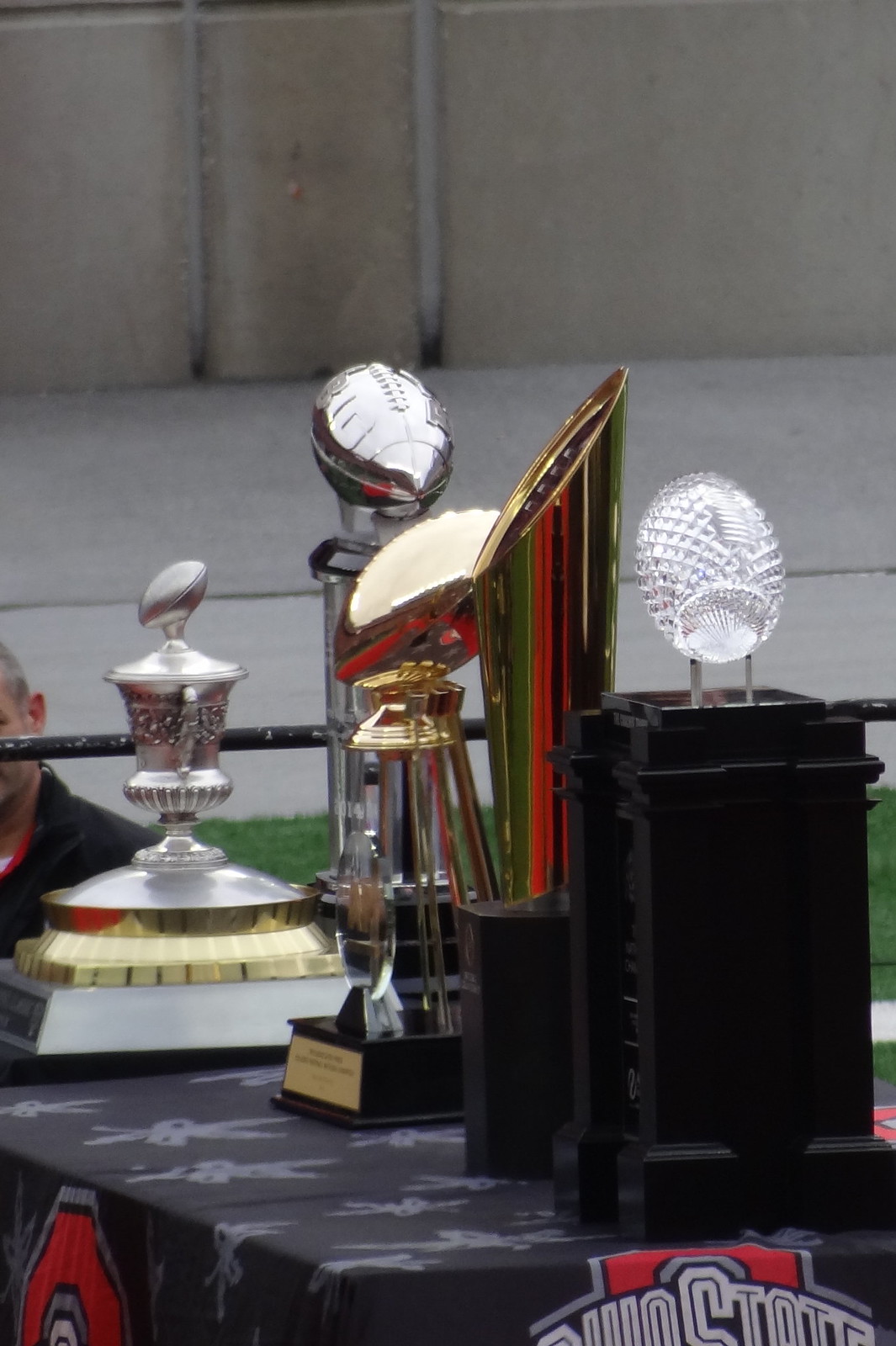This detailed photograph, taken at an indoor venue, showcases five distinct football trophies arranged on a rectangular table. The table is draped with a black and grey cloth, prominently featuring an Ohio State logo in red and grey across the front and side, although the accompanying text is obscured. The background reveals a green surface that might be lawn or astroturf, along with white walls and a ceiling marked by horizontal and vertical lines. A metal handrail is visible on the left, behind which a man's head and shoulders can be partially seen.

The trophies exhibit a variety of designs:
1. A cup with a rugby ball on a large base.
2. A larger trophy also featuring a rugby ball.
3. A gold trophy with a rugby ball on top.
4. A trophy resembling the trumpet part of a tuba.
5. A black rectangular plinth topped with a crystal rugby ball.

Together, these elements suggest a possible setting for an Ohio State event, perhaps a press conference, where their collection of football trophies is on display.